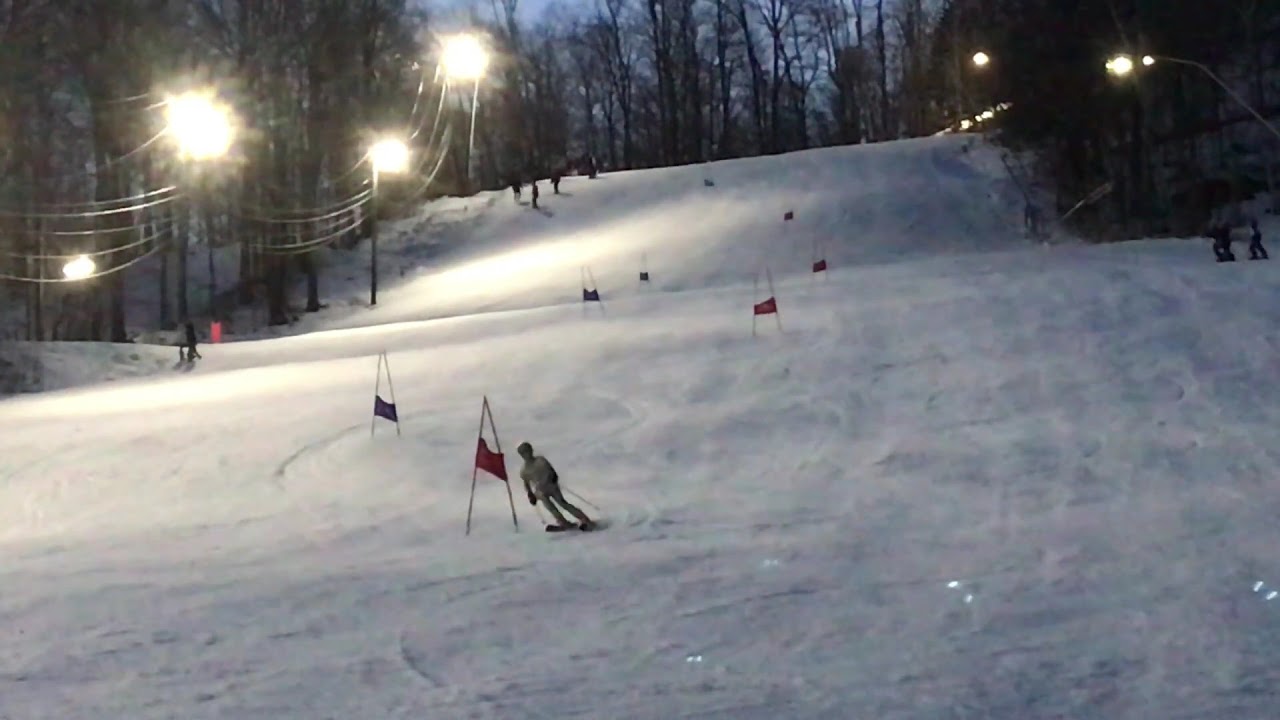The image captures a scenic ski slope just as the evening begins to set in. The wide expanse of the snow-covered slope is adorned with red and green flags, possibly marking the course for skiers. The scene is illuminated by numerous lights that delineate the slope and hint at the oncoming darkness, though a touch of daylight remains visible in the sky. A solitary skier glides down the snowy expanse, their features indistinct from the distance. Surrounding the slope on either side are sparse, leafless trees, their bare trunks standing out against the snow. In the distance, the slope inclines upward to meet a higher hill, where more bare trees punctuate the horizon, outlining the serene, wintry landscape.